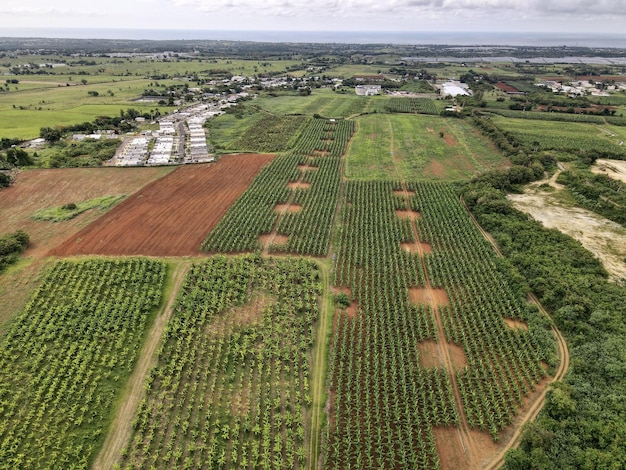This aerial photograph showcases a vast agricultural landscape characterized by diverse fields and a serene ambiance. Dominated by fields of various crops, some distinctly identifiable as corn, the scene captures an intricate patchwork of agricultural activity. Interspersed among these cultivated areas are sections of barren earth, possibly indicating resting fields or freshly tilled soil. The middle section is conspicuously composed of fields with irregular shapes, enhancing the picturesque quality of the landscape.

To the right, a river gracefully winds through the scenery, adding a fluid element to the otherwise static croplands. Adjacent to this river, some areas of dense shrubbery and a murky green pond are visible, contributing to the varied textures within the image. On the periphery, a mobile home park and a housing complex can be seen, along with several scattered buildings that might serve as storage facilities or perhaps dwellings for the local community.

In the distant background, the photograph reveals a thin strip of clouds hovering above what seems to be the ocean or gently rolling coastal hills, suggesting a location likely in central coastal California. The cloudy sky casts a peaceful, subdued light over the entire scene, encapsulating the tranquil essence of rural life.